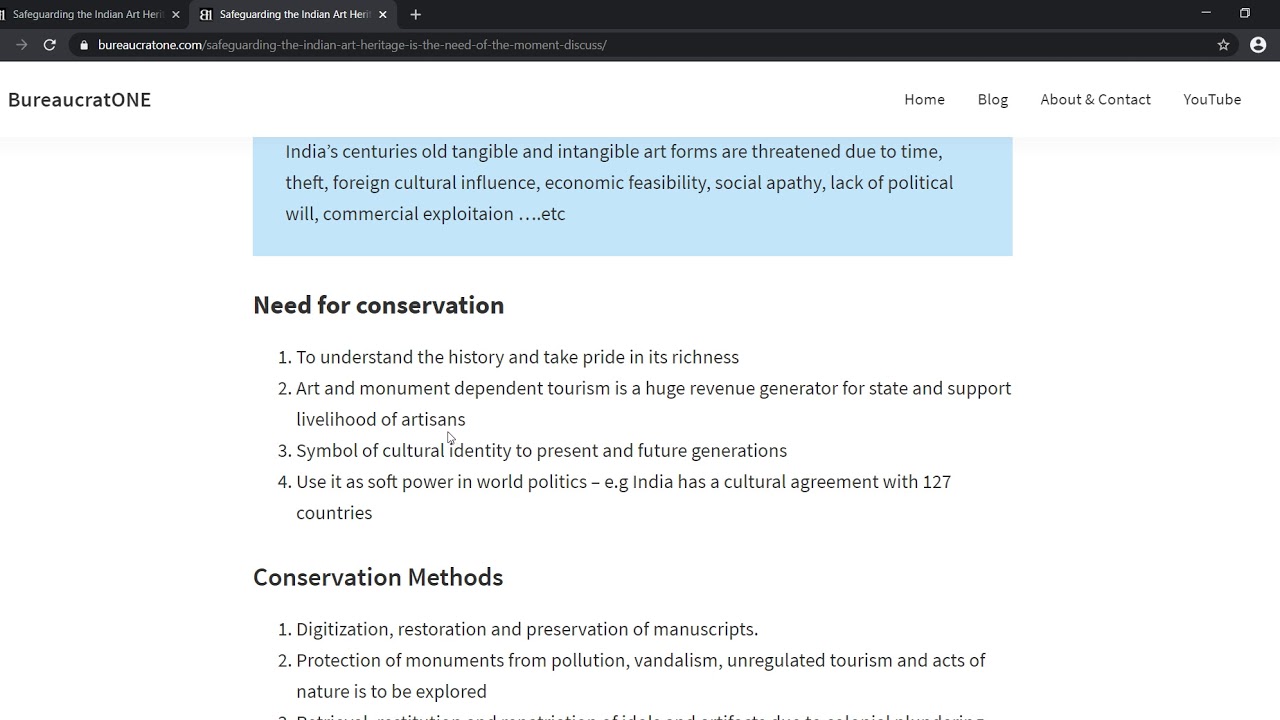A screen displaying the website Birokhash.com appears, foregrounded by multiple navigation elements including 'Home,' 'Blog,' 'About,' 'Content,' and 'YouTube.' Dominating the background is a blue square with the text: "India's Centuries-Old Tangible and Intangible Art Forms," highlighting the foreign cultural influences, economic visibility, social apathy, and commercialization challenges these arts face. The message emphasizes the necessity for conservation to understand India's historical richness and instill pride. It notes that tourism based on art and monuments generates significant state revenue and supports artisans' livelihoods. Art is portrayed as a symbol of cultural identity crucial for future generations and as a tool for soft power in global politics. It mentions India's cultural agreements with 127 countries and lists conservation methods including digitization, restoration, and protection of manuscripts and monuments from threats like pollution, vandalism, unregulated tourism, and natural disasters. The website appears dedicated to a bureaucratic mission with links to a Home page, Blog, Facebook, Twitter, and YouTube.